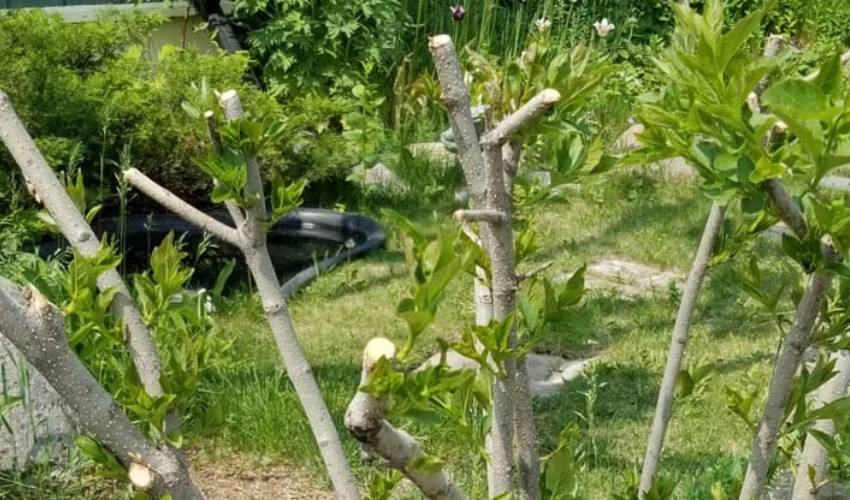This vibrant color photograph depicts a meticulously maintained backyard that showcases the efforts of an avid gardener. Central to the image are several pruned trees with thick, white trunks from which branches extend upward, freshly cut at their tops and midsections. From these blunt and clean-shaven branches, fresh foliage is beginning to regrow. The trees, numbering around six or seven, are surrounded by a lush carpet of green grass interspersed with other greenery, including tall grasses, weeds, and patches of exposed dirt at the bottom of the image.

A stone path, sparsely laid, meanders behind these pruned trees. On the left side of the path lies a small pond, contributing to the serene garden ambiance. In the background, clusters of white flowers and tall grasses can be seen, enhancing the garden's natural beauty. Also visible in the photograph's far left is a mysterious black object, though its identity is uncertain. The photo angle appears to be slightly above ground level, capturing the entire scene without any people or animals, focusing solely on the greenery and garden elements.